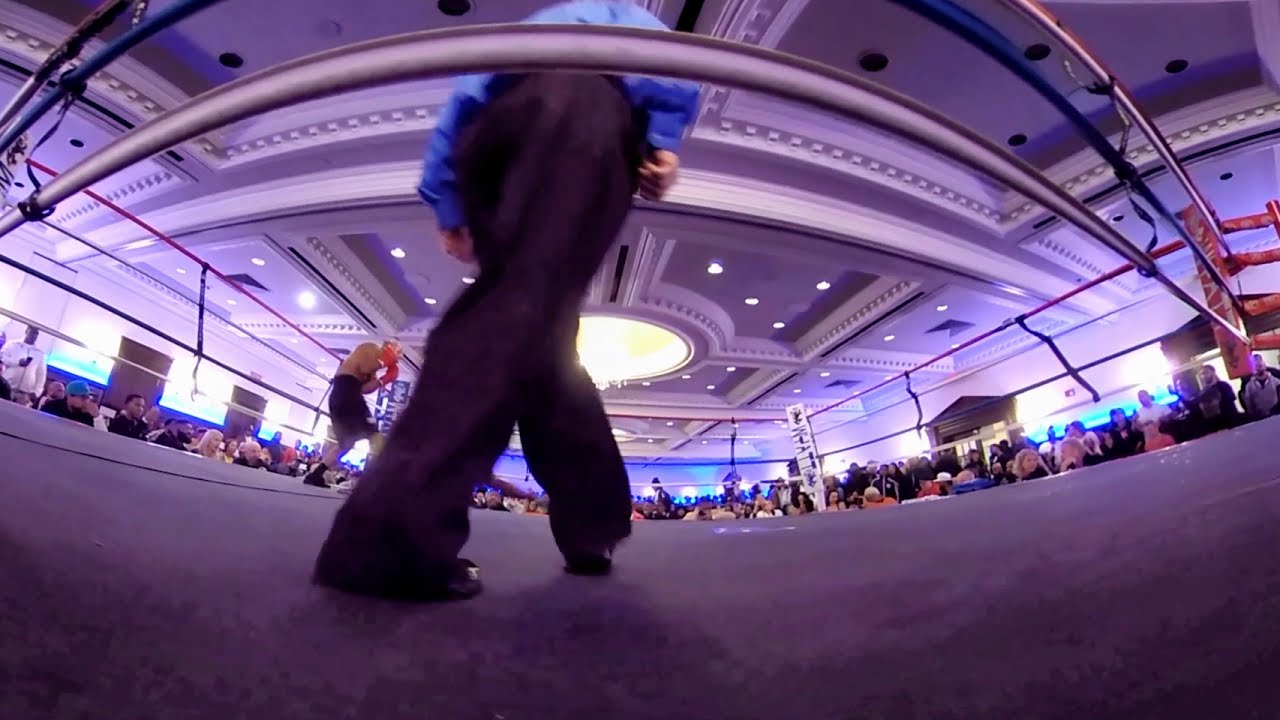A distorted wide-angle photograph captures the scene from the floor level of a boxing ring, providing a unique perspective. The image is taken from outside the ring, just below the ropes, which are colored red, blue, and white. The back of a referee dominates the foreground; he is attired in black pants and a blue t-shirt, his hands visible, and stands near the bottom ropes with his legs and lower torso prominently in view. To the left, farther inside the ring, a boxer with red gloves raises his hands, dressed in black shorts, socks, and shoes, his shirtless torso slightly bent forward and turned away from the camera. Surrounding the ring is a crowd of spectators, their presence evident on all sides. The ceiling above suggests an unexpectedly grand venue for a boxing match, adorned with ornate wainscoting, intricate moldings, support beams, recessed lights, and a central chandelier, hinting at the elegance of a banquet hall.